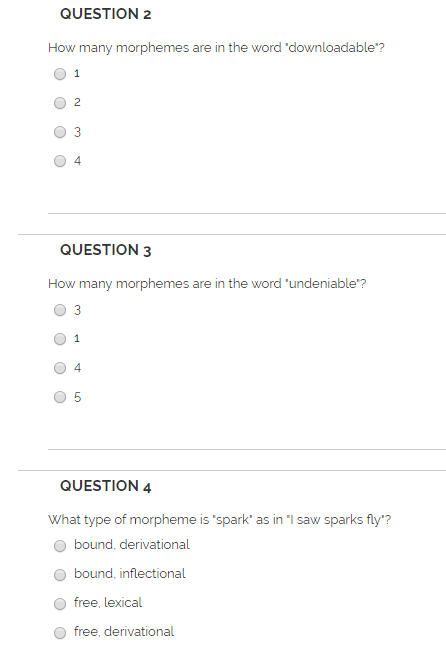The image appears to be a section of a linguistic test or quiz with a clear, white background and dark black text for the main questions. 

In the top left corner, in a bold black font, "Question 2" is stated. Directly beneath, in a lighter font, the question reads: "How many morphemes are in the word 'downloadable'?" with a question mark at the end. Below this question are four circles, each paired with a number ranging from one to four.

Below "Question 2", there are two black dividing lines followed by "Question 3" in the same bold black font. The accompanying question in lighter text reads: "How many morphemes are in the word 'undeniable'?" This question is followed by a set of four circles again, but this time the options are labeled as three, one, four, and five.

Following another set of two black lines, "Question 4" appears in bold black text. The question in lighter font asks: "What type of morpheme is 'spark' as in 'I saw sparks fly'?" Below this question, there are four circles with the following options: 
1. Bound, derivative 
2. Bound, inflectional
3. Free, lexical (notable spelling error: "lexiv")
4. Free, derivational (indicating a notable mispronunciation: "deratumeral").

This concludes the visible content on the page, which exclusively consists of these three questions. The speaker expresses their difficulty with English and a humorous self-awareness about their performance on the test.